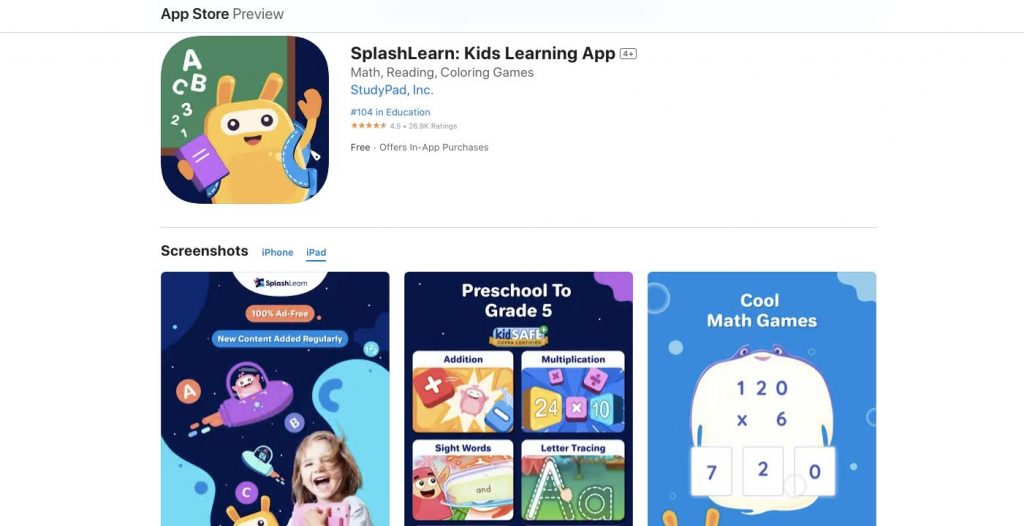On a clean white background, the image prominently features the title "App Store Preview" in black on the upper left side. Beneath it, there is a small, detailed thumbnail icon of the app; it depicts a cheerful yellow creature wearing a blue backpack and holding a book, standing in front of a green chalkboard with "ABC123" written on it in white chalk.

To the right of this thumbnail, the text "SplashLearn Kids Learning App 4+, Math, Reading, Coloring Games" is displayed in black. Below this, "StudyPad Inc." is listed in blue, along with the ranking "#104 in Education" also in blue. Adjacent to this, a yellow star rating is displayed, showing an impressive "4 1⁄2" stars based on 26.9K ratings, and indicating that the app is free with in-app purchases available.

Underneath these details are three vibrant, colorful screenshots from the app. The first screenshot on the left shows a smiling child in front of a cartoon background, accompanied by the app's yellow creature character in a spaceship. The middle screenshot has a dark, minimalistic background with white text that reads: "Preschool to Grade 5, Addition, Multiplication, Sight Words, Letter Tracing." The third screenshot on the right has a blue background showcasing the image of a cartoon stingray, viewed from its white-bellied underside, which is marked with the multiplication problem "120 x 6" and its solution "720."